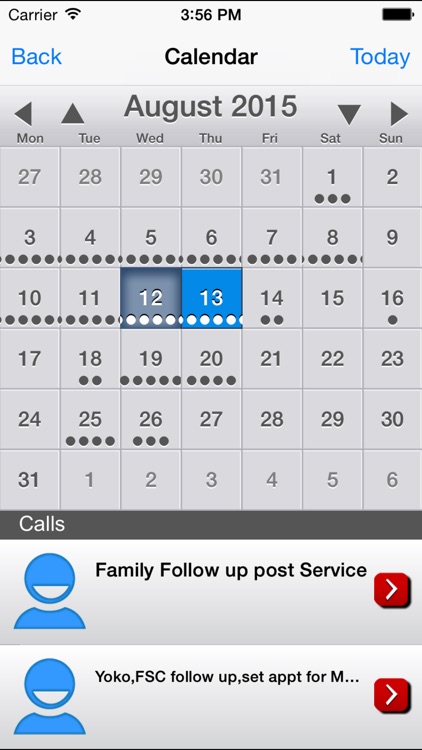The image is a screenshot of a smartphone calendar app, captured on August 2015. In the top left corner, the screen displays the carrier information and a Wi-Fi signal icon, followed by the time, which reads 3:56 p.m., and a full battery indicator to the right. Below this, there's a blue 'Back' button on the top left and a 'Today' button on the far right. The header reads "Calendar."

The main display shows the calendar of August 2015, with selected dates marked by dots: 1, 3, 4, 5, 6, 7, 8, 10, 11, 12, 13, 14, 16, 19, 20, 25, and 26, likely indicating special events or reminders. Highlighted are the dates 12 and 13, with the 12th marked in dark gray and the 13th in blue, suggesting a particular focus on these days.

At the bottom of the screen, there are call-to-action prompts with buttons. The first prompt states "Family follow-up post service" with a red button beneath it, and the second one reads "Yoko FSC follow-up set appointment for," also accompanied by a red button.